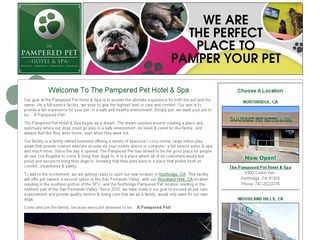The image features a multifaceted design centered around pet care services. On the upper left section, there is a green background with a white circle that encloses a stylized green dog paw, notable for its unique three-pad design. Below this emblem, the text "Pampered Pet Hotel & Spa" is prominently displayed. 

In the middle, the upper portion showcases a charming image of a bulldog alongside another dog, set against a vibrant blue, pink, and green background. Below the dogs, in bold black text, the statement "We are a perfect place to pamper your pet" is clearly visible.

Further down, there is a paragraph that begins with "Welcome to Pampered Pet Hotel & Spa" in gray text, followed by an extensive amount of much smaller gray text that is illegible due to its diminutive size in the context of the photo.

On the right side of the image, there's a photograph of the Pampered Pet Hotel & Spa building, distinguished by its tan exterior. A partial view of another location appears beneath this picture, but it is cut off and incomplete.

This comprehensive image aims to promote the Pampered Pet Hotel & Spa, blending visual and textual elements to convey a message of luxury and care for beloved pets.